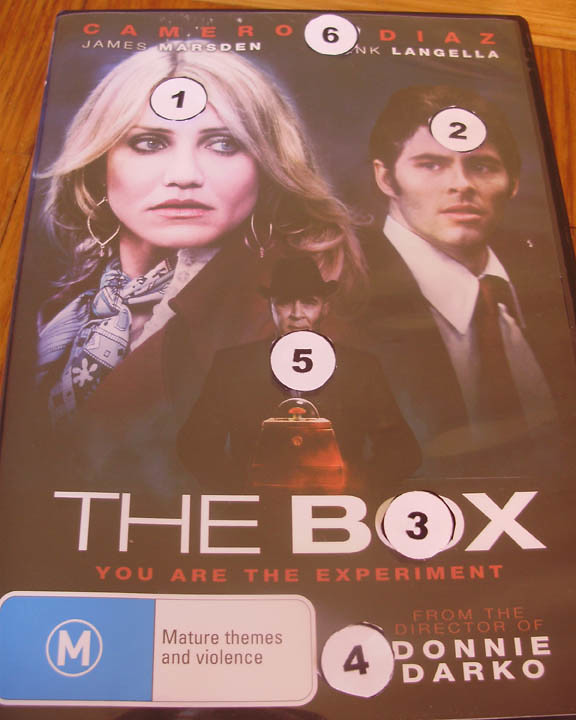This image depicts a DVD box set of the movie "The Box," which is laying on a wooden table. The cover is in color and prominently features the names of the lead actors: Cameron Diaz, James Marsden, and Frank Langella, arranged across the top. Cameron Diaz appears significantly on the left side of the cover, wearing a scarf and designer jacket; she is a white actress with blonde hair. To her immediate right is James Marsden, a white actor with brunette hair, dressed in a suit and tie. Positioned centrally between them is Frank Langella, holding a box.

Numbered stickers are placed over different elements on the cover:
- A '1' is on Cameron Diaz's forehead.
- A '2' is on James Marsden's head.
- A '3' is near the movie title.
- A '4' is near the text mentioning the director of "Donnie Darko."
- Frank Langella has a '5' over him.
- A '6' is over the collection of names at the top.

The movie’s title, "The Box," is boldly printed at the bottom of the cover in large, white text, followed by the subtitle "You are the Experiment." The phrase "From the director of Donnie Darko" is also prominently displayed on the bottom right. Additionally, a white "M" enclosed in a circle with a blue background, indicating mature themes and violence, suggests a foreign rating system. The movie is based on an episode of the reimagined "Twilight Zone" series from the mid-1980s.